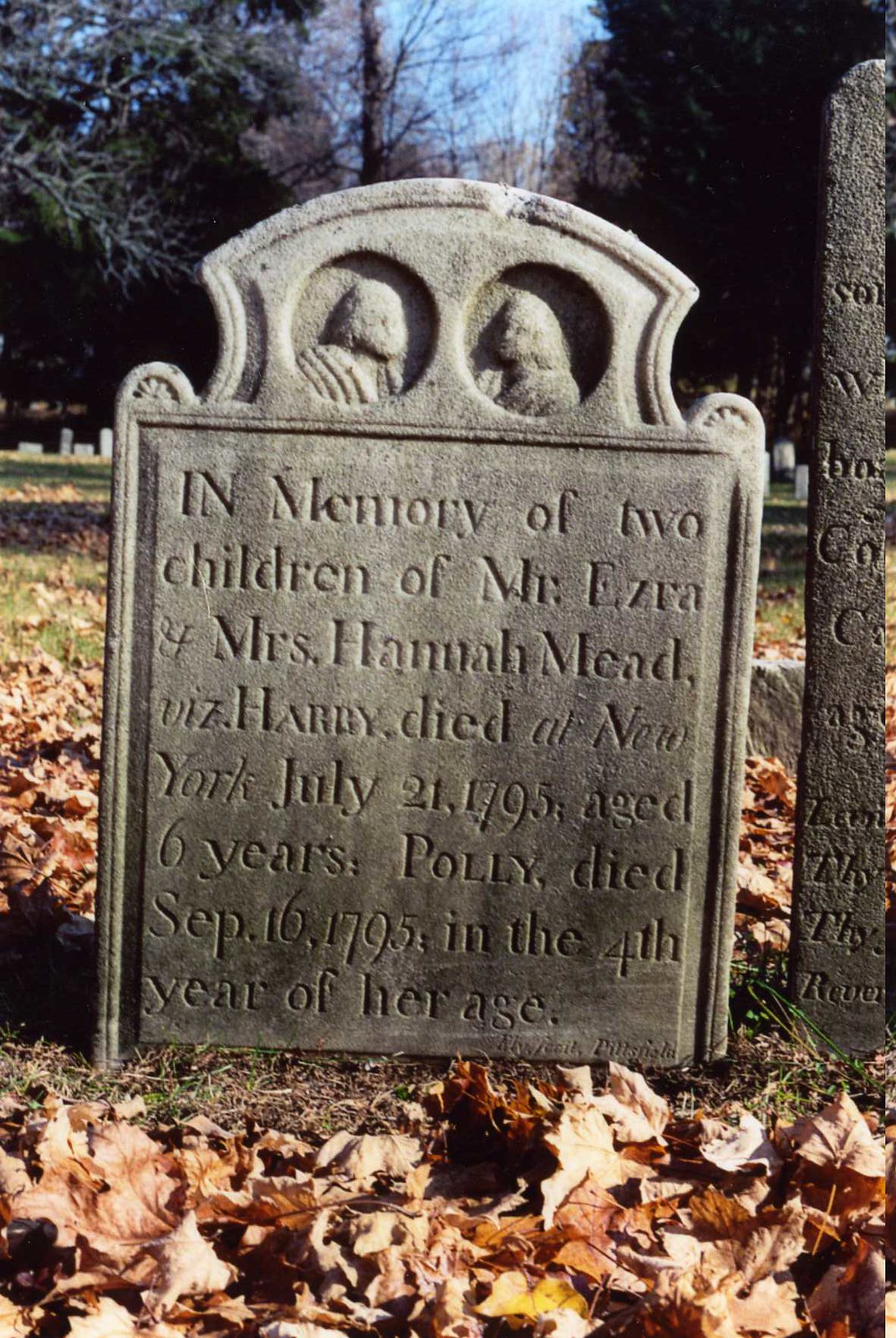Amidst the serene autumn landscape, an intricate gravestone stands solemnly in a graveyard, surrounded by a scattering of fallen leaves. This close-up shot reveals a memorial dedicated to two children of Mr. Ezra and Mrs. Hannah Mead. The inscriptions poignantly recount that Harry died in New York on July 21, 1795, at the tender age of 6, while Polly passed away on September 16, 1795, in the fourth year of her life. The gravestone, crafted from concrete, is adorned at the top with delicate carvings of two children placing their hands tenderly, symbolizing the innocence and purity of the departed. To the right of this gravestone, a smaller, timeworn stone with barely legible text stands in quiet companionship. In the background, lush cedar trees punctuate the view, along with glimpses of other gravestones, offering a glimpse into a bygone era.